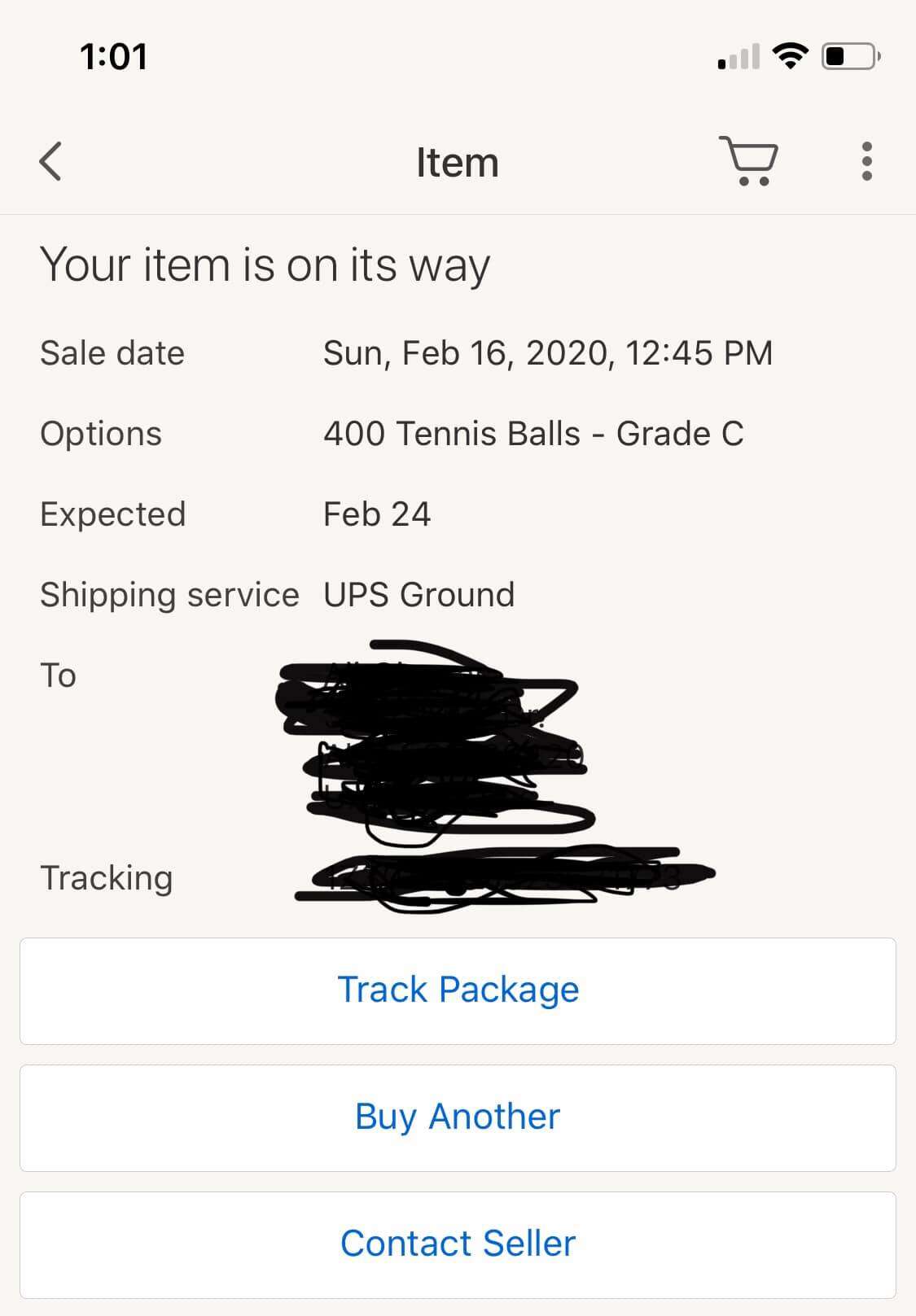Here is a cleaned-up and detailed caption for the described image:

---

A digital screenshot taken from a smartphone displays a transaction confirmation screen. At the top, the device shows the time as 1:01 PM along with a battery icon indicating roughly 25% charge remaining, and WiFi signal bars. Below the status bar, there is a section labeled "Item" accompanied by a shopping cart icon and three gray dots, indicating a menu or options.

The message "Your item is on the way" is prominently displayed. The purchase details include:
- **Sale Date**: Sunday, February 16, 2020 at 12:45 PM
- **Options**: 500 tennis balls, Grade C
- **Expected Delivery Date**: February 24
- **Shipping Service**: UPS Ground

Following the purchase information, there is a "To" section which includes the delivery address and recipient's name, both of which have been blacked out for privacy.

At the bottom, there are action buttons labeled "Track Package," "Buy Another," and "Contact Seller." The overall color scheme includes white and blue.

---

This reformulated caption provides a structured and clear description of the screenshot content.